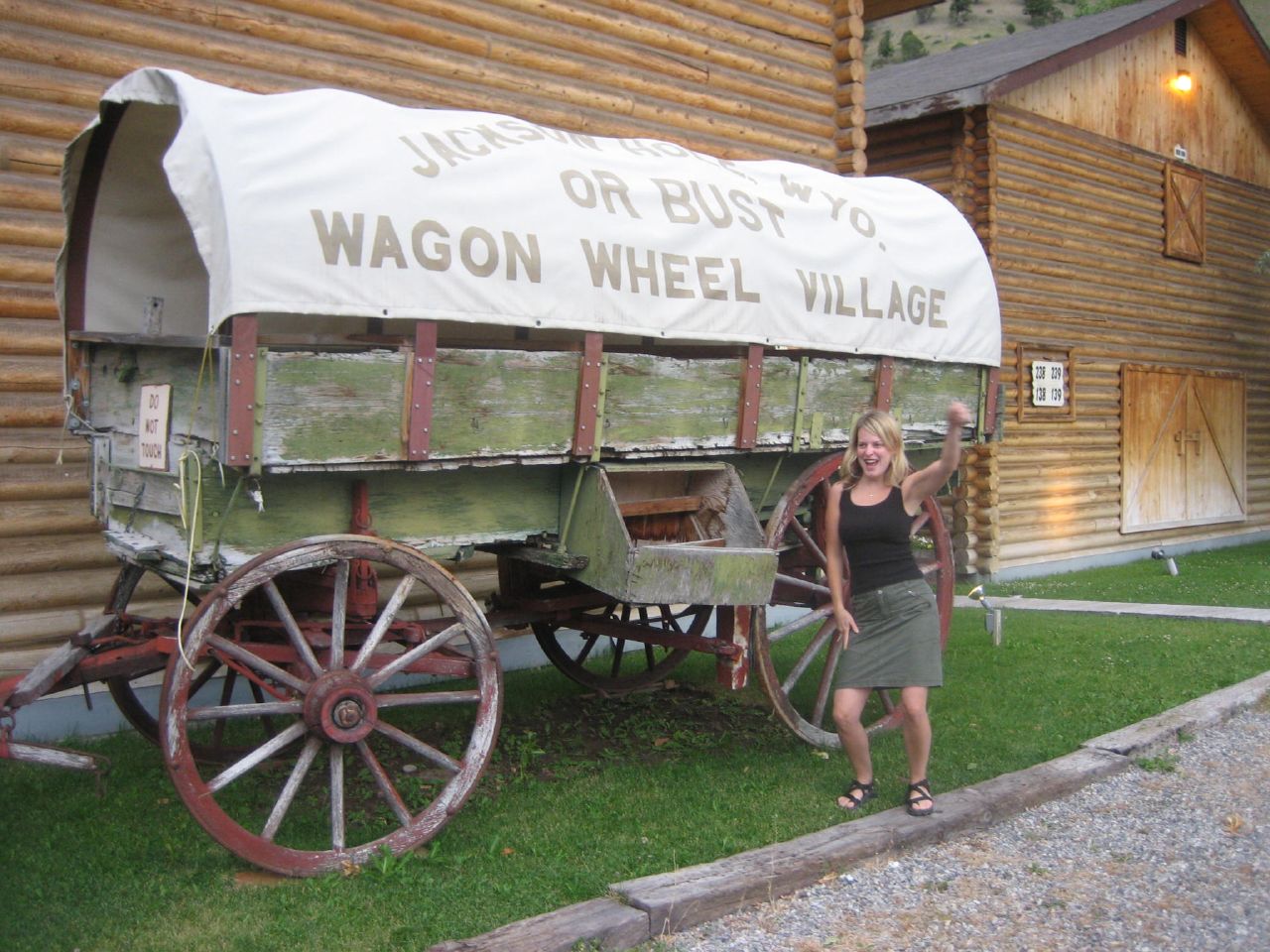In this detailed outdoor daytime scene, we see a vibrant and nostalgic display of an old Western-style village. Central to the image is a lively woman with shoulder-length blonde hair, wearing a sleeveless black tank top, a gray skirt, and black sandals. Striking a playful pose, she has her left arm raised in a circular motion as if lassoing something, and her right arm resting on her thigh, her mouth open as if exclaiming "yee-haw."

Directly behind her is an old-fashioned wooden covered wagon, painted green but now weathered with chipping paint revealing gray patches. The wagon features red wheels and a white canvas tarp, which reads "Jackson Hole, Wyoming or Bust Wagon Wheel Village." Surrounding the wagon is a grassy field that extends into the background, where two-story log cabins stand tall. These log cabins, with their sloping gray roofs, boast square brown shutters on their double doors and singular windows positioned centrally on their upper stories.

To the foreground and lower right, a gravel road is lined with large square lumber pieces, possibly railroad ties, adding to the rustic charm of the scene. The entire setting evokes a sense of historic Americana, capturing the essence of a picturesque old town village display.